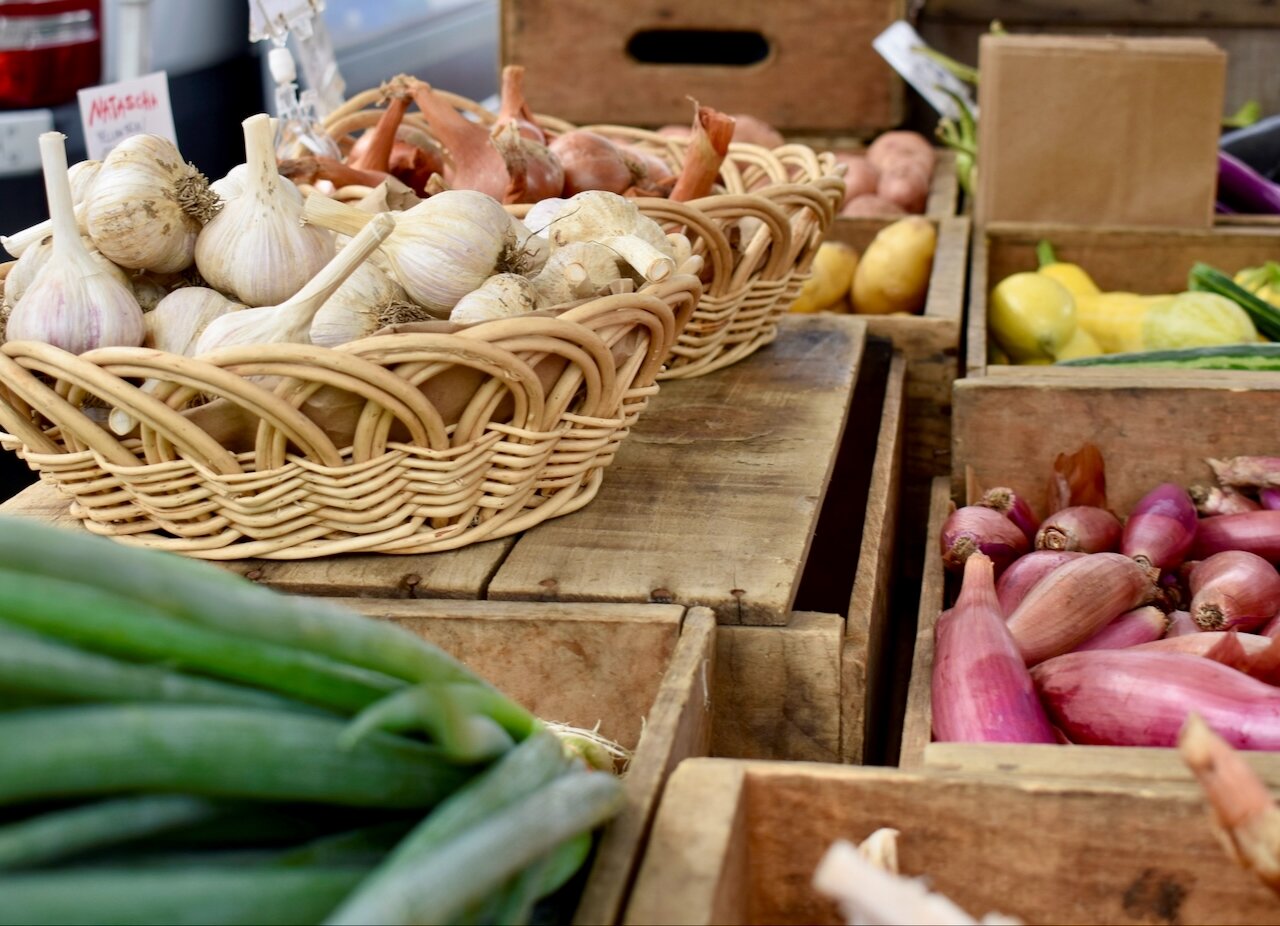The photograph captures an outdoor produce display, evident from the partial view of a vehicle's tail light in the background. The produce is meticulously arranged in woven wicker baskets and weathered wooden crates, showcasing a variety of vegetables. Two wicker baskets prominently feature garlic bulbs—white garlic in the foreground and more brown-shaded garlic in the background. Other visible produce includes yellow squash, potatoes, red shallots, and both green and red onions, with some ambiguity surrounding additional vegetables that might be eggplants or snap peas. Small, out-of-focus paper signs are tucked into the garlic baskets and other areas, hinting at labels or prices but remaining illegible. The photorealistic image emphasizes the texture and arrangement of the vegetables against the rustic backdrop of aged crates.